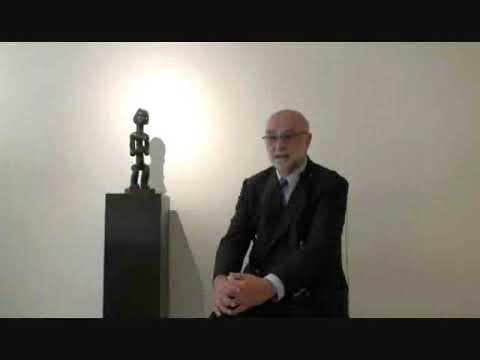The image features an older white male, approximately 60 years old, sitting indoors. He is bald and wears glasses, with a white beard giving him a distinguished appearance. Dressed in a formal black suit, accompanied by a white shirt and a black tie, he appears quite official. His legs are crossed, and he rests his hands, fingers intertwined, on his knee. To his right, a tall, rectangular black pillar supports a metal-colored statue of a small human figure. The background is predominantly white, and there is a noticeable illumination, possibly from a camera flash. At the bottom of the image, yellow text on a black background reads, "During the last 50 years, they had a lot of stock which...," an incomplete statement hinting at a historical context. The overall scene exudes a sense of formality and significance.